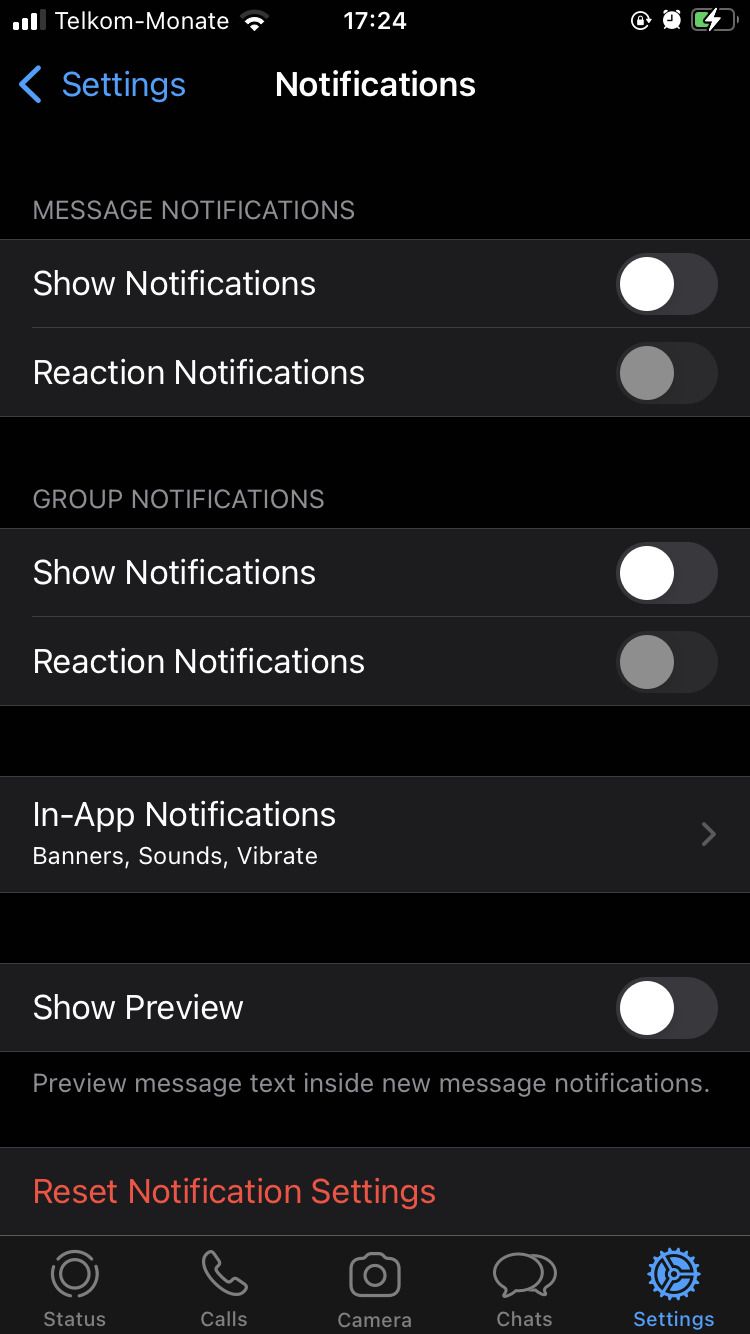This is a detailed screenshot from a mobile phone's notification settings. The top section of the screenshot has a black background with white text, displaying various status indicators. From left to right, you can see the mobile signal icon followed by the text "telecom/monate," a Wi-Fi icon, the time shown as 17:24, an alarm clock icon, and a battery icon.

Below this status bar, the background transitions to white with text in different colors. In the top-left corner in purple font, it reads "Settings," accompanied by a left-pointing arrow. Beside it, in white font, it says "Notifications."

Further down, in gray font, it reads "Message Notifications," followed by two gray rectangular buttons with white text. The first button says "Show Notifications" and the second says "Reaction Notifications," both of which feature toggle switches set to off.

Continuing down, it says "Group Notifications" in gray font, again followed by "Show Notifications" and "Reaction Notifications," both with toggles also set to off.

At the bottom in white font, it reads "In-App Notifications," followed by three descriptors: "Banners," "Sounds," and "Vibrate." Below this, it says "Show Preview" in white font, accompanied by a toggle switch also set to off.